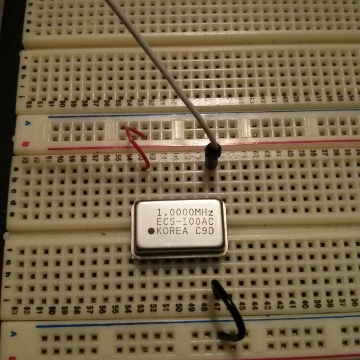The square color photograph captures a close-up view of an ivory-colored electronic component. This component is composed of rectangular, grid-like segments reminiscent of a stretched-out ice cube tray, with each containing tiny square holes arranged in a precise pattern—five rows of twenty columns. Along the short side of the rectangles are labeled sequences of letters A, B, C, D, E, F, while the long side features numbers, which seem to span from the 60s downward, suggesting the component extends significantly beyond the visible section in the photograph. Various metallic details populate the component: some squares have small metallic hooks and wires, including a noticeable black wire looping between squares and a red wire similarly connected between points. A significant feature of the image is a silver metallic rectangle inscribed with detailed specifications: "1.0000 MHz, ECS-100AC, Korea, C9D." The section in view highlights the meticulously organized and labeled structure typical of such electronic pieces.